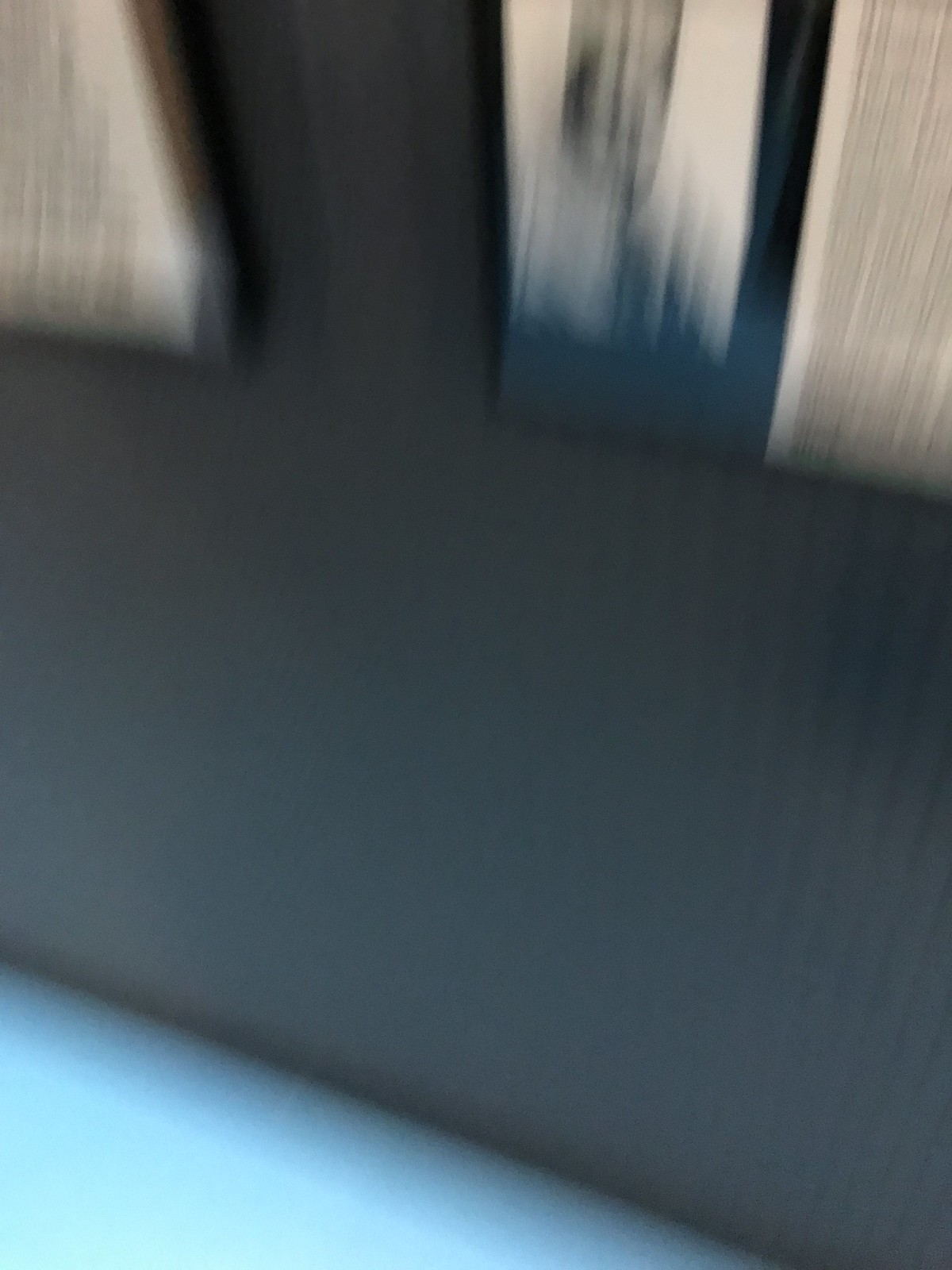This photograph captures a scene featuring a dark charcoal gray wall adorned with two black-framed items, which may be plaques or posters. Due to the blur in the image, details are indistinct, but each frame appears to contain a photograph on the left side and text on the right, possibly commemorating an individual or event. The floor is a light blue color, contrasting with the darker hues of the wall and frames, adding a subtle but noticeable touch to the composition.